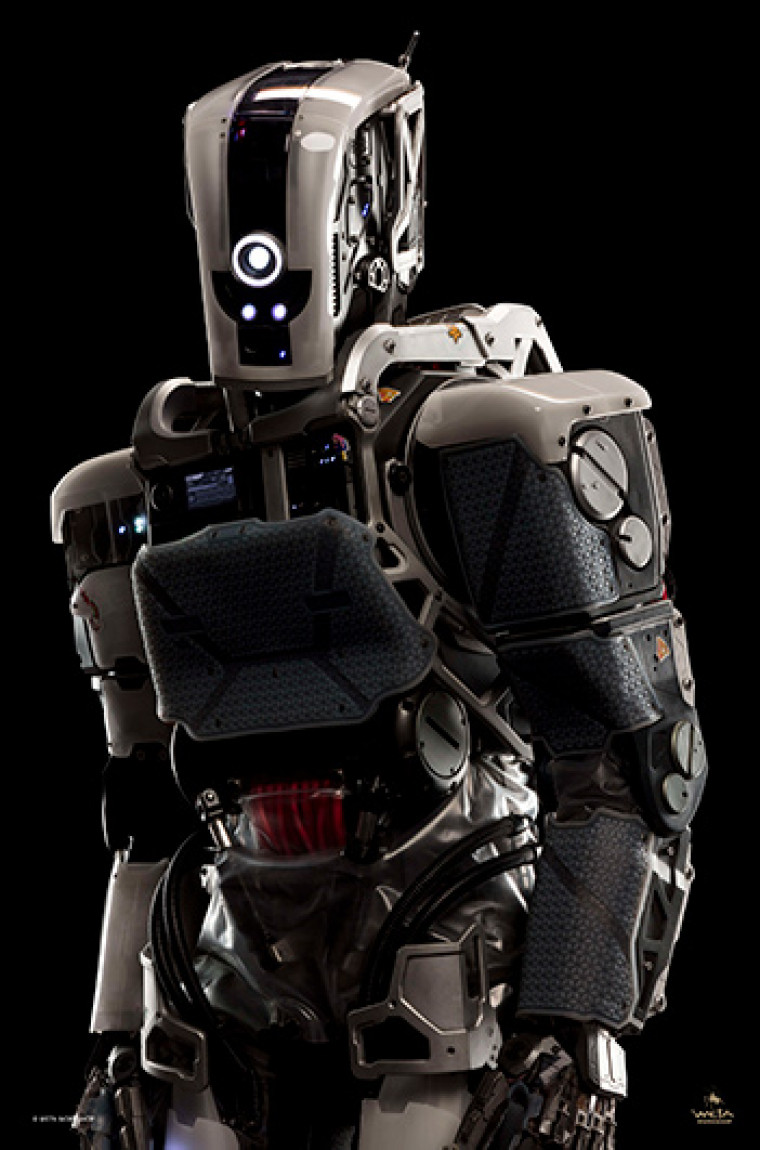This photograph showcases a human-like cyborg set against a black background, crafted predominantly from metal and an array of mechanical components. The cyborg's overall color palette includes shades of brown, cream, black, and hints of orange. It features a robust robotic frame, complete with distinct mechanical arms and legs that match the creamish hue of the body. The cyborg's head is sizable and composed of a composite material, akin to a desktop computer tower with a prominent white power button in the center. Dominating its face is a singular luminescent eye in the middle of its head, accompanied by two smaller circles that might also serve as eyes, though their function is unclear. Red wiring is visible throughout its inner structure. The chest of the cyborg houses a black speaker-like box and is complemented by large, squared shoulders that appear reinforced with metal shoulder pads, adding to its striking and intricate design.